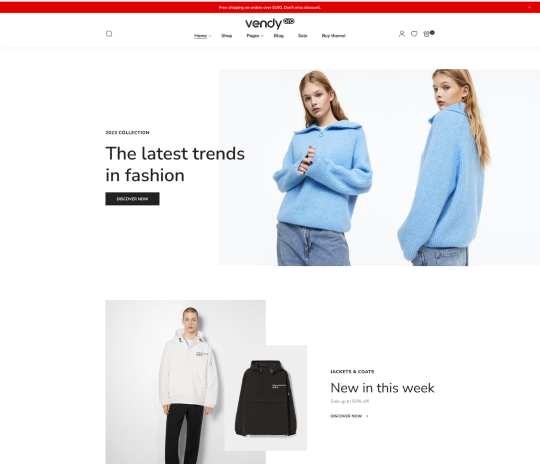The image is a screenshot of a web page from a fashion retail website called "Vendy." The layout is predominantly white, giving it a clean and modern look. A striking red stripe runs horizontally from the upper left corner to the upper right corner, adding a pop of color to the interface. Centered below the stripe is the bold text "Vendy," spelled out as V-E-N-D-Y, indicating the brand name. Beneath this header, there are several tab categories for site navigation.

On the left, there is a sidebar labeled "The Latest Trends and Fashions," which lists current fashion updates. This sidebar blends seamlessly into the main content area, where various images of models showcase different outfits. 

The first model is a light-skinned woman with blonde hair, pictured in two shots. In the first shot, she faces forward and dons a blue sweater. In the second, taken from a profile angle, she wears the same blue sweater while facing left.

Below these images, another model—a light-skinned man—appears, wearing a large white hoodie paired with black pants. Adjacent to this, there is a separate image of the same hoodie in black.

To the far right of the screen, text reads "New in This Week," emphasizing the website's commitment to offering the latest fashion trends. Vendy appears to be a dynamic and constantly updated platform, ensuring shoppers have access to the newest clothing options available.